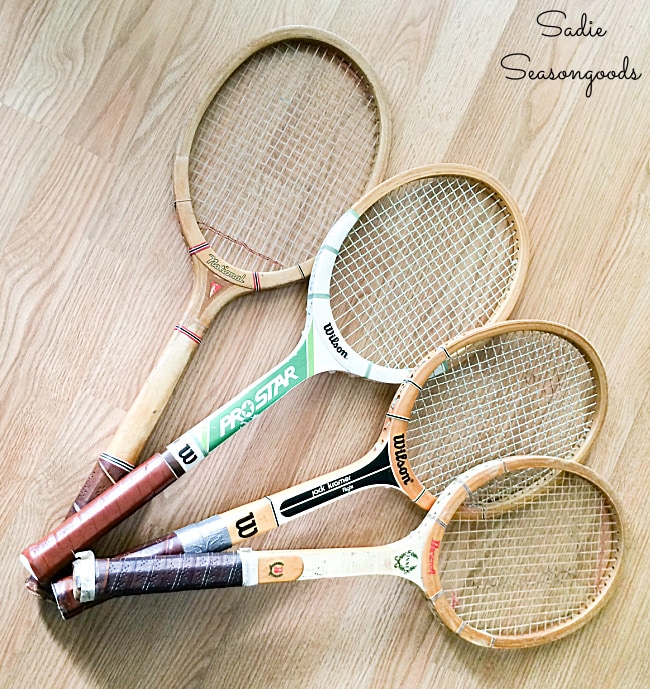This meticulously curated photograph captures four vintage wooden tennis rackets artfully displayed in a fan formation on a light wood paneled floor, highlighting the organic texture and grooves of the floorboards. Each racket, characterized by its white strings and brown leather-wrapped handles, showcases unique details yet they all exude a classic Wilson brand aesthetic. From left to right: the first racket features a tan handle; the second has a maroon handle with "Pro Star" in green text along with a blue "W" tape on the frame; the third is characterized by a brown handle and partially blue detailing with a black "W" logo; and the fourth, distinct with its white neck, rests horizontally across the others. Completing the image, in the upper right corner, the phrase "Sadie Seasonal Goods" is elegantly inscribed in black cursive script, adding a refined touch to this vintage-themed composition.